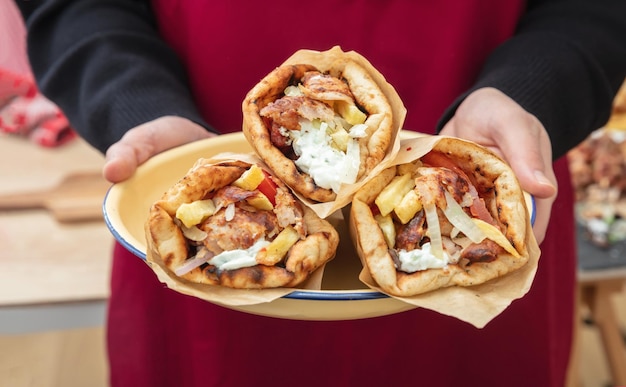In this landscape-oriented color photograph, the focus is on a person holding a shallow yellow bowl with a blue painted rim, positioned mid-chest to mid-hip. The individual, wearing long black sleeves and a dark red apron, extends their hands to present the bowl towards the viewer. Inside the bowl are three neatly wrapped gyros, showcasing beige pita shells with browned edges, wrapped in brown butcher's paper. The open ends of the gyros face the viewer, revealing thinly sliced grilled meats - chicken on the top left and bottom, steak pieces visible on the right, generously slathered with white tzatziki sauce, and accompanied by chopped tomatoes and other ingredients. The background features a counter with various out-of-focus items, including a cutting board, assorted ingredients, brown meat on the right, and what appear to be towels or oven mitts towards the top left. The meticulous details and vibrant presentation highlight the appetizing nature of the food, captured in a realistic and representational style of food photography.